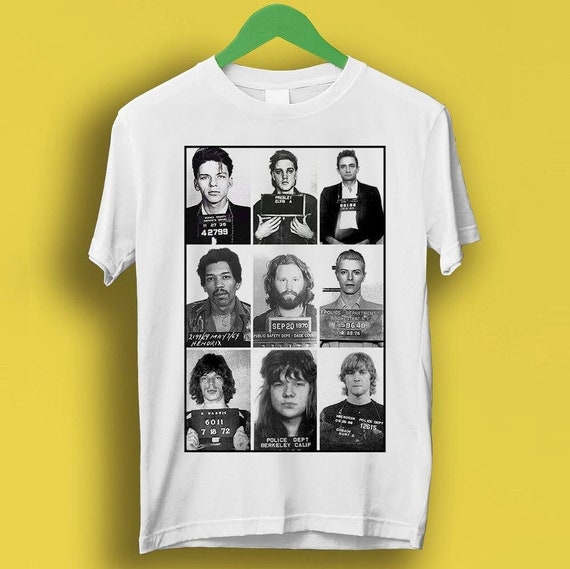This image features a white short-sleeved t-shirt hanging on a green hanger against a yellow background. The focal point of the t-shirt is a grid of nine black-and-white mug shots, organized into three rows of three. Each photograph displays the face of a well-known musician, depicted from the chest upwards, with prison numbers visible beneath some of the images. The top row features Frank Sinatra, Elvis Presley, and Johnny Cash from left to right (our perspective), while the middle row includes Jimi Hendrix, Jim Morrison, and David Bowie. The bottom row showcases Mick Jagger, Janis Joplin, and an unidentified young male that may resemble Kurt Cobain. This striking design combines iconic imagery of famous musicians with a uniform presentation, creating a visually engaging tribute to these legendary figures.